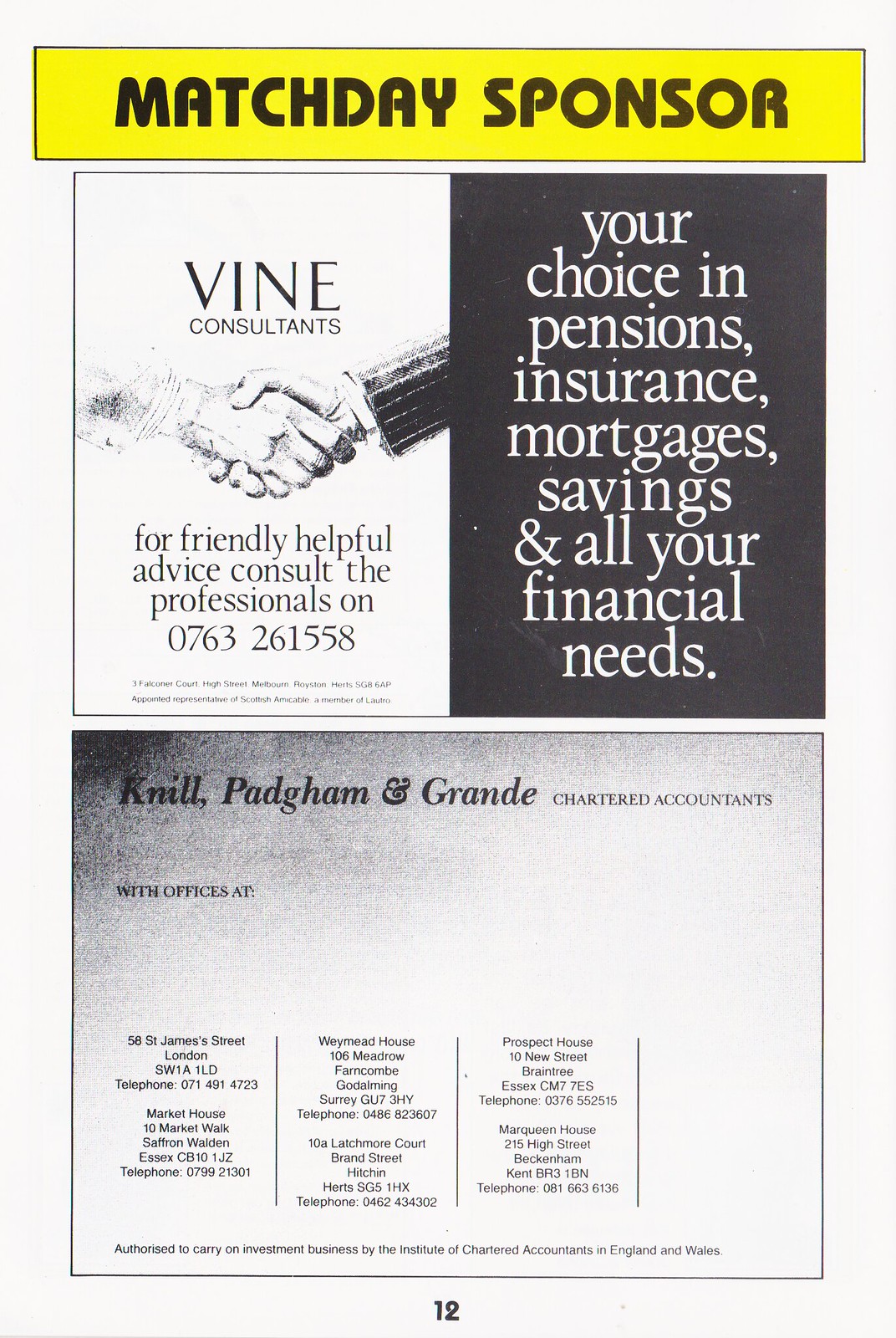This magazine page features an advertisement with a white background. At the top, there is a narrow yellow rectangle with black text that reads, "Match Day Sponsor." Below this, on the left side, against a white background, there is black text that reads, "Find Consultants for Friendly Helpful Advice, Consult the Professionals," followed by a phone number. An illustration of two hands shaking, implying a business agreement, accompanies this text. On the right side, with a contrasting black background, white text reads, "Your Choice in Pensions, Insurance, Mortgages, Savings, and All Your Financial Needs." 

The bottom half of the page returns to a white background with some shadowy black in the upper corner. This section contains black text that reads, "NIL, PAGAM, and Grande, Chartered Accountants, with offices at St. James Street, London, WeMed House, Prospect House," providing details of the chartered accountants' office locations and contact information.